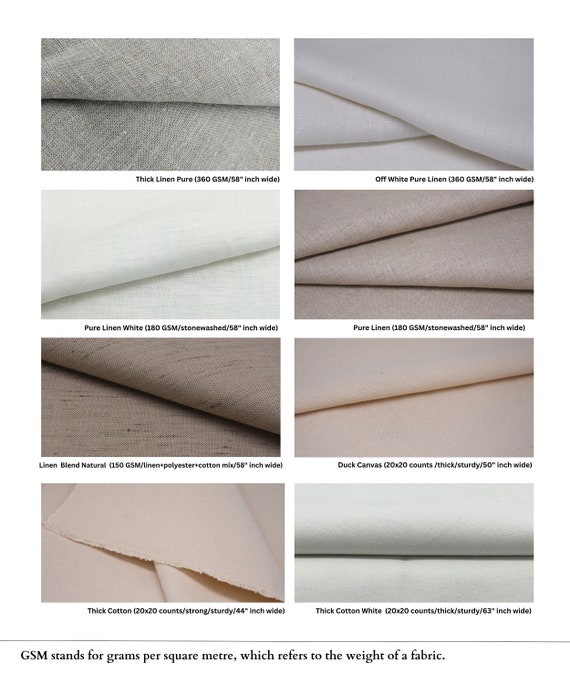The image resembles a catalog page displaying eight different fabric swatches, arranged in two columns and four rows, each labeled with detailed specifications. On the top left, there's a thick pure linen fabric, gray with small white patterns, rated at 360 gsm and 58 inches wide. Directly to its right, the top right image shows an off-white pure linen fabric, also at 360 gsm and 58 inches wide. Below the gray linen on the left, there's a pure white linen fabric, stonewashed and weighing 180 gsm at 58 inches wide, while to the right of it is a light brown stonewashed pure linen fabric of the same weight and width.

The third row begins with a natural-colored linen blend fabric featuring a brown base with black dotted patterns; it's a mix of linen, polyester, and cotton, weighing 150 gsm and measuring 58 inches wide. Adjacent to this on the right, a light pink fabric labeled as duck canvas, with a composition rating of 20 x 20 counts and a sturdy texture, 50 inches wide. On the bottom left, there's another light pink fabric, a thick cotton rated at 20 x 20 counts and 44 inches wide. The last swatch on the bottom right is a white thick cotton fabric, 20 x 20 counts, and the widest among the cottons at 63 inches. A footnote at the bottom clarifies that gsm stands for grams per square meter, referring to the fabric's weight.